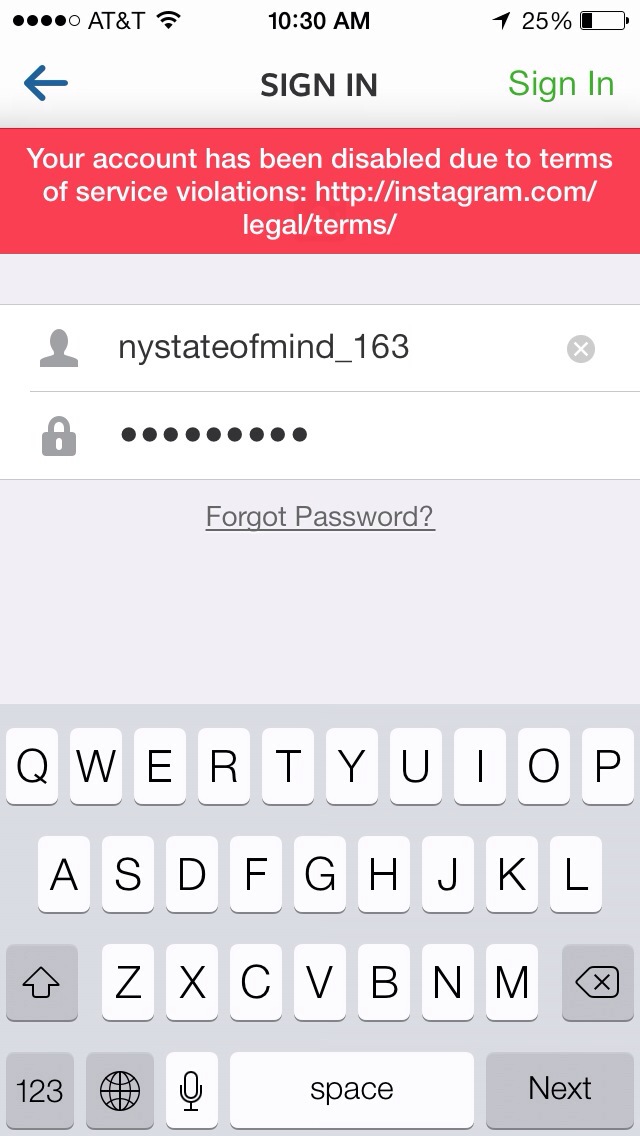The image is a vertical screenshot from an iOS device, showing a disabled social media account warning from Instagram. At the very top, the status bar reveals that the carrier is AT&T, the time is 10:30 AM, and the battery level is at 25%. Centered below, the title reads "Sign In," with a green link on the right and a back button on the left. 

A conspicuous red banner informs the user with the message, "Your account has been disabled due to terms of service violations," followed by a link to Instagram's terms of service: http://instagram.com/legal/terms. 

Below the banner, the username "nystateofmind_163" is displayed with password fields filled with obfuscated dots. There's a link below these fields that reads "Forgot password?" At the very bottom of the screenshot, a keyboard is displayed, featuring a QWERTY layout without numbers. The keyboard includes a microphone symbol and a world globe symbol to the left of the space bar. The overall composition uses a color scheme of red, white, black, gray, and green, and the image is structured with the status and alert at the top, followed by input fields and the keyboard at the bottom.